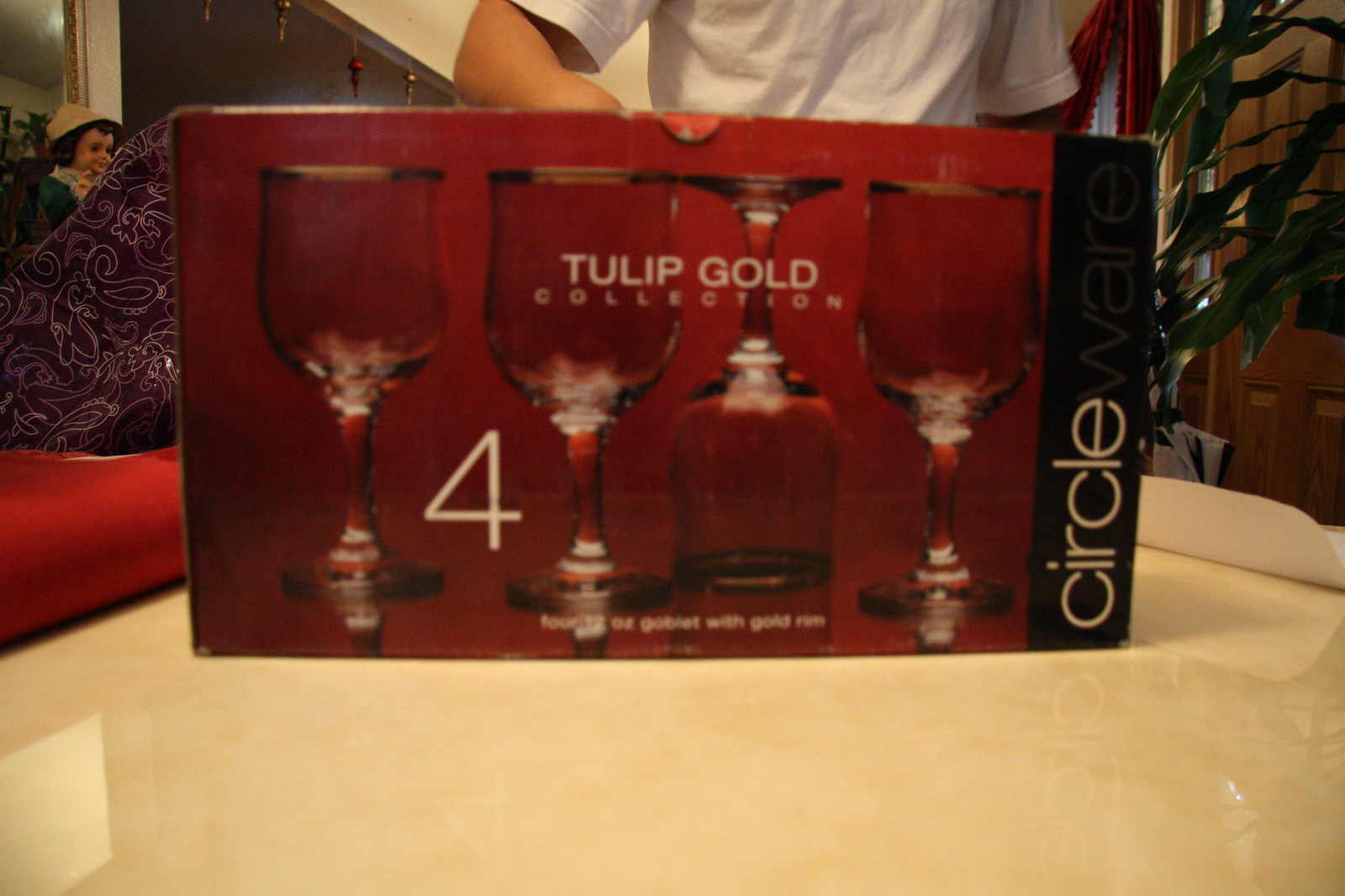The photograph features a close-up of a red rectangular box prominently placed in the center on an off-white, marble-like table. The box displays an image of four goblet-style wine glasses: the first two upright, the third upside down, and the fourth upright again. Bold text on the box reads "TULIP GOLD" with "COLLECTION" beneath it. A number "4" is located in the left corner, while a black vertical strip on the right-hand side includes the words "CIRCLE WEAR" in white letters. Behind the box, a person in a white short-sleeved t-shirt is partly visible, showing only their chest area and slightly raised left arm. In the background, to the left of the person, is a small doll dressed in a green outfit and sporting a wicker bonnet, alongside various purplish and red materials. To the right, a large plant with long, upward-pointing leaves peeks out from behind the box.